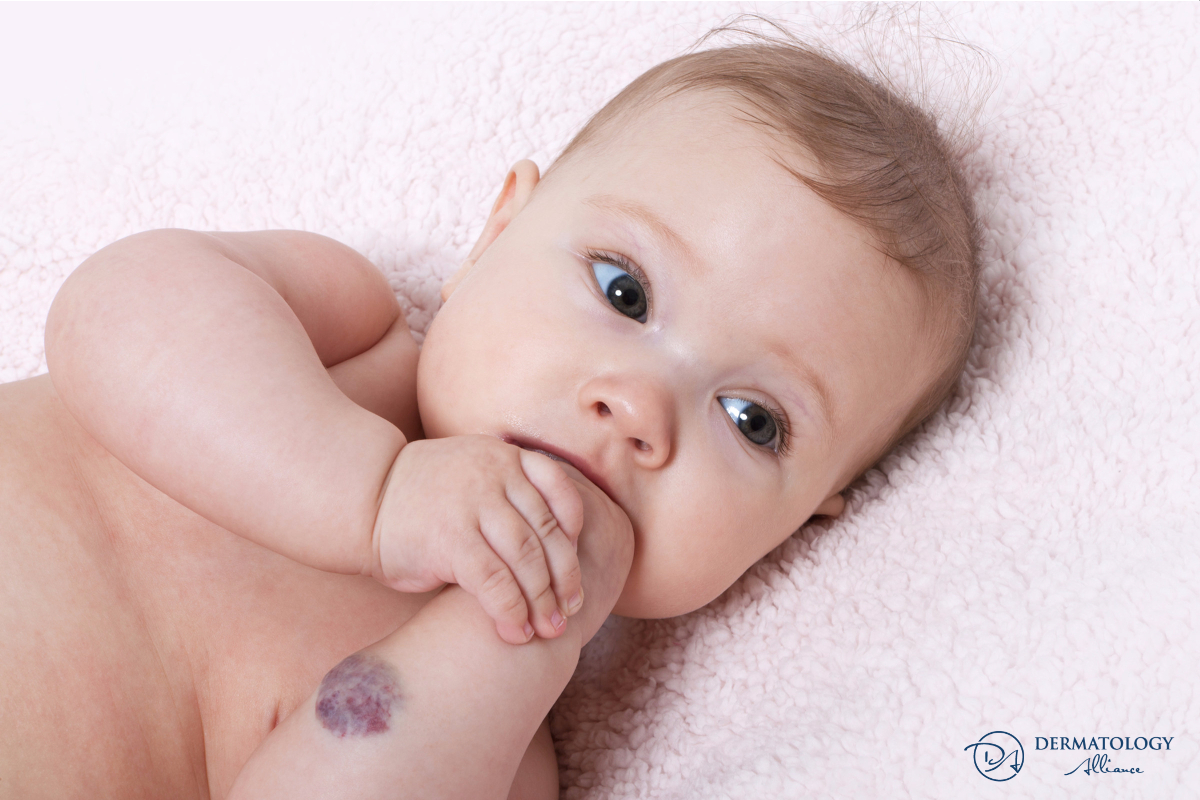In the photograph, we see a close-up, color image of an infant lying diagonally on a plush, white fuzzy blanket. The baby is shirtless, displaying the top half of its body with a slightly wavy, dark blonde fuzz of hair and big, open blue eyes looking off to the right. The infant has its left hand in its mouth, while its right hand grasps the left wrist. There's a noticeable, round, purplish mark that could be a bruise or a birthmark on the baby's left forearm. In the bottom right corner of the image, there is a watermark logo in a circle with the initials "DA" and the text "Dermatology Alliance" underneath, indicating that this image is part of an advertisement for a dermatology clinic.